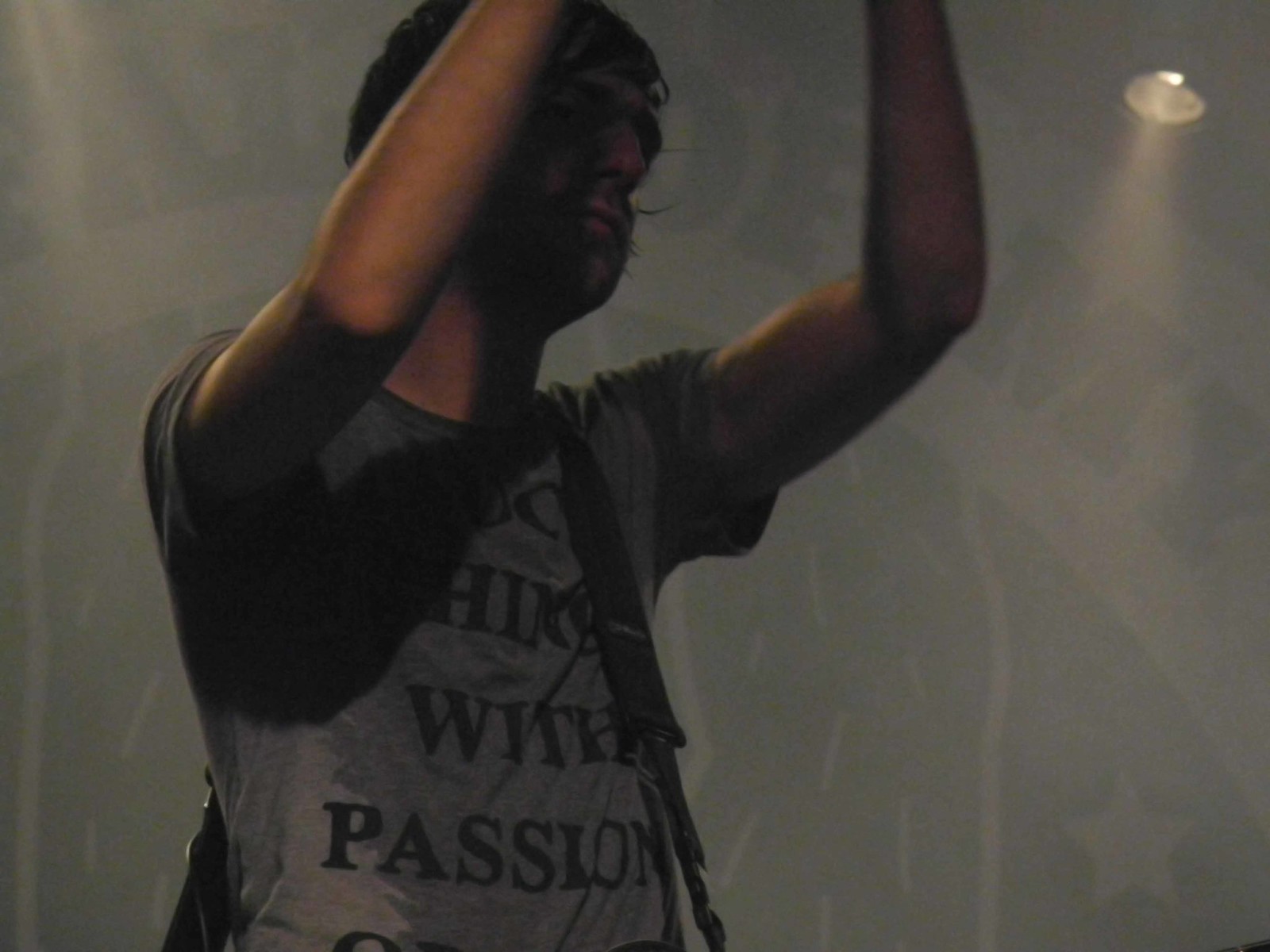The image is a realistic, possibly photographic depiction of a man, who might be a musician performing at a concert. Centered slightly to the left in the frame, the man faces right at an angle with both arms raised, disappearing out of the image above the wrists. He has medium-length, shaggy, dark-colored hair, and wears a gray t-shirt featuring black lettering. The shirt appears to be sweat-stained or wet, with more distinct darker areas in the middle. The visible text includes the words "with passion," though the rest is unclear or partially obscured. A black strap, likely for a guitar, runs across his left shoulder. His face is mostly in shadow, contributing to a tired or solemn expression. The background is dark, featuring a faint, unidentifiable image and a light in the upper right corner. Some additional faint elements such as a star might be discernible in the bottom right-hand corner.